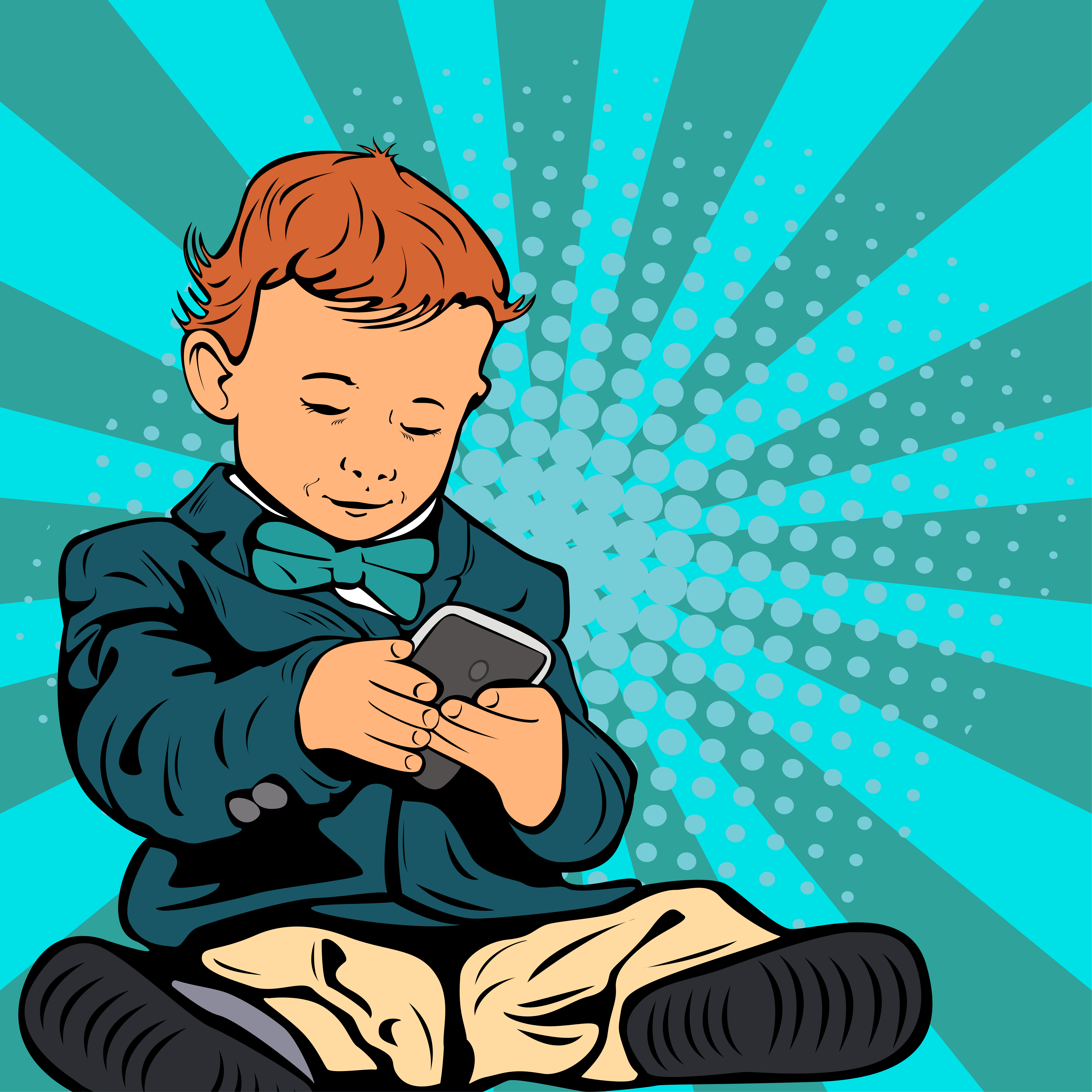In this detailed digital artwork, a charming toddler with auburn-red hair and fair skin sits engrossed in a black smartphone. His hair has a few upturned cowlicks and curls at the sides, adding a playful touch to his look. He is dressed in a blue-green suit jacket paired with a lighter green bow tie, complemented by khaki-colored pants. The jacket is slightly crinkled and marked with dark lines that highlight its bends. The bottoms of his black shoes, showing their tread pattern, are visible as his legs are splayed out. The boy, appearing to be around two or three years old, wears a look of deep concentration as he studies the smartphone in his hands. Adding to the whimsical feel of the scene, the background is an explosion of vibrant color, featuring alternating green and dark green rays with overlying geometric green circles packed together towards the center. The overall piece evokes a vintage 1950s cartoon style, combined with a contemporary pop art aesthetic, creating a striking and quirky visual experience.